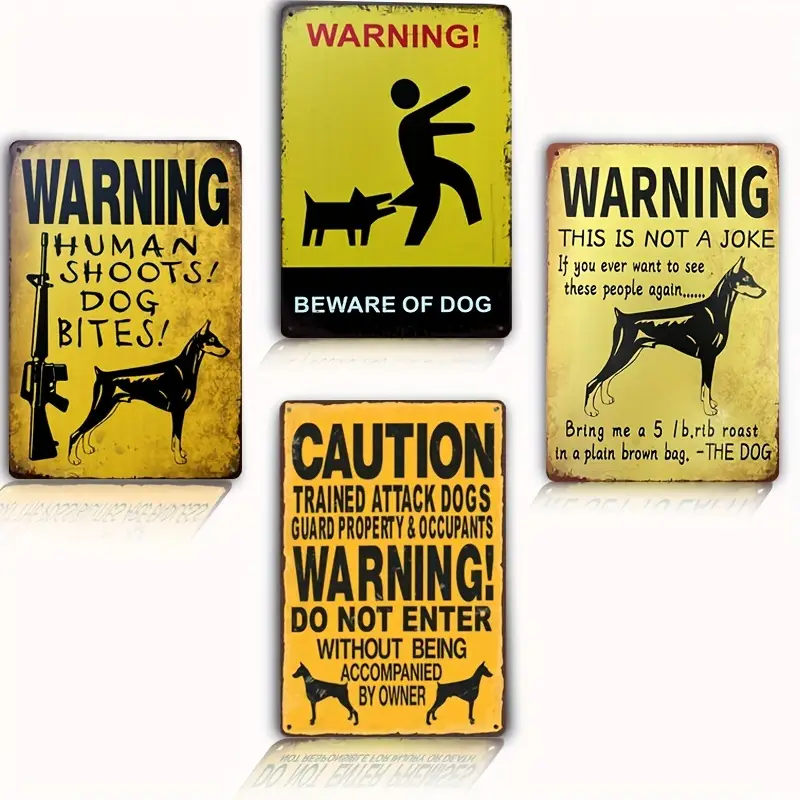Four metal signs with varying shades of yellow and black text hang in a linear arrangement against a white background. Each sign serves as a warning about dogs. The first sign, positioned on the left middle, states, "Warning: Human shoots, dog bites," featuring a Doberman Pinscher facing right and a machine gun with its barrel pointing up. Directly above in the top middle, another sign reads, "Warning: Beware of Dog," and depicts a stick figure with a dog biting its rear; notable for its red warning text and a distinctive black bar at the bottom. The third sign, on the right middle, humorously warns, "Warning: This is not a joke. If you ever want to see these people again, bring me a five-pound rib roast in a plain brown bag. - The Dog." The final sign, found at the bottom, declares, "Caution: Trained attack dogs guard property and occupants. Do not enter without being accompanied by the owner," and features illustrations of two Rottweilers.